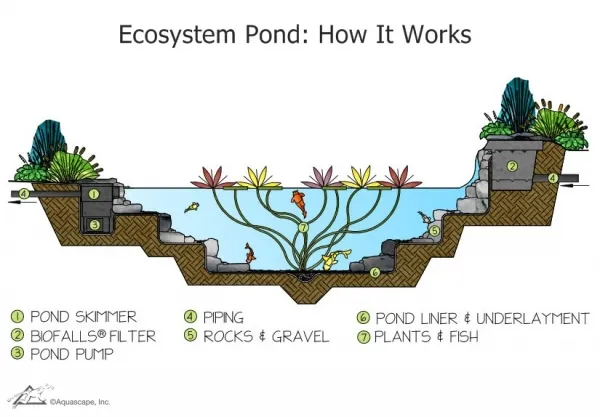This vibrant, colored illustration diagram titled "Ecosystem Pond: How It Works" is displayed prominently at the top of the page. The cross-section of the pond shows a detailed and colorful ecosystem with numerous elements labeled for clarity. The surface of the pond is adorned with lilies, various green plants, and rocks on the top left and right sides, while the water teems with numerous fish. Tendrils from a flowering plant at the bottom of the pond stretch upwards, blooming into red, yellow, and pink flowers. The pond has multiple steps and layers, highlighted by key components like the pond skimmer, biofalls filter, pond pump, and piping. Rocks and gravel, pond liner and underlayment, and various plants and fish are numerically labeled 1 to 7. Each part of the pond is intricately connected, with detailed descriptions below the diagram. The bottom left corner features a small illustration of a frog within a triangle, marked with "Copyright Aquascape Incorporated." This detailed depiction serves as an informative guide to understanding the complex workings of an ecosystem pond.